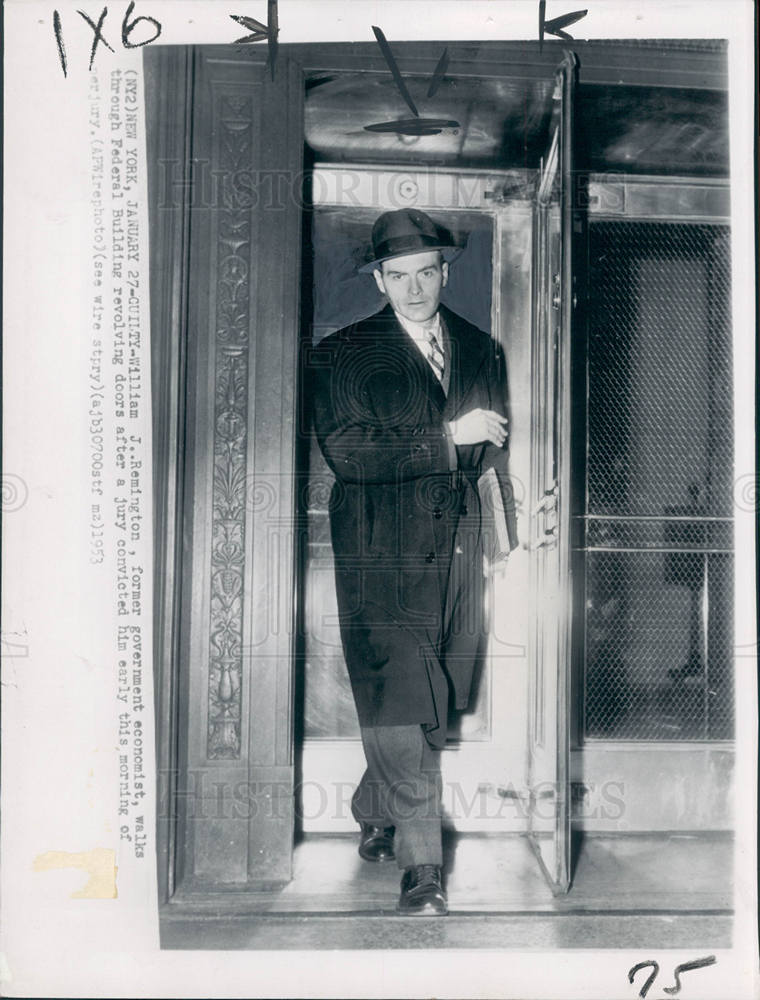This black-and-white photograph, watermarked with "Historic Images" at the top and bottom, captures a serious-looking man, identified as William J. Remington, a former government economist, walking out of a federal building's revolving doors. Remington is dressed in a dark trench coat over a suit, with a black top hat, a black-and-white striped tie, and gray pants. He carries a book or folder tucked under his left arm while using his right hand to push the revolving door. Notably, there is a visible number "75" in the bottom right corner of the image and "1 x 6" written in the top left corner. The caption inscribed on the photograph reads: "New York, January 27th. Guilty. William J. Remington, former government economist, walks through the federal building revolving doors after a jury convicted him of perjury early this morning."